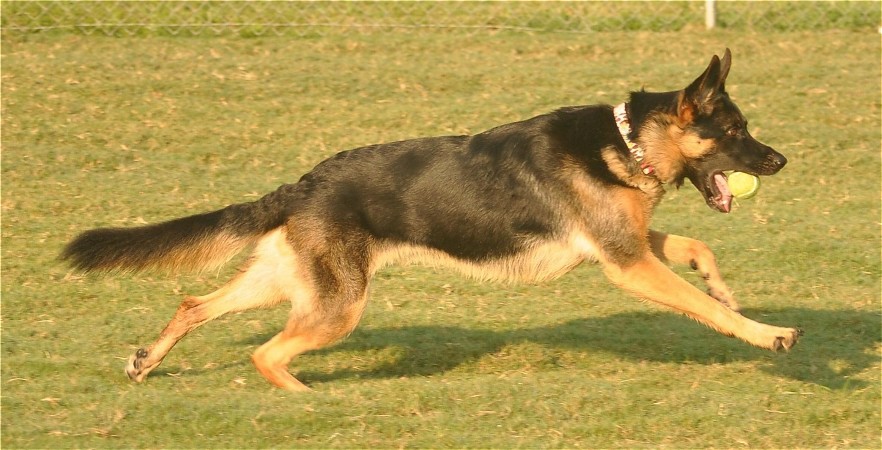This vibrant outdoor photograph captures the dynamic moment of a German Shepherd in mid-gallop, running to the right in a large, freshly trimmed grassy yard. The dog, positioned centrally in the image, has a striking black-and-tan coat: his back, face, ears, and the top of his tail are a dark black, while his legs, paws, and part of his body exhibit a rich tan hue. He sports a colorful collar and his mouth is wide open, proudly carrying a yellow tennis ball. One of his paws touches the ground while the others are airborne, highlighting the intensity of his playful run. At the very top of the photograph, the outline of a traditional metal chain-link fence is faintly visible, adding a subtle boundary to the expansive yard. Scattered across the green grass are brown leaves or helicopter seeds, enhancing the natural, lively setting of this action-packed scene. The German Shepherd's brown eyes and black nose are discernible, adding to the vivid detail of this joyful moment.